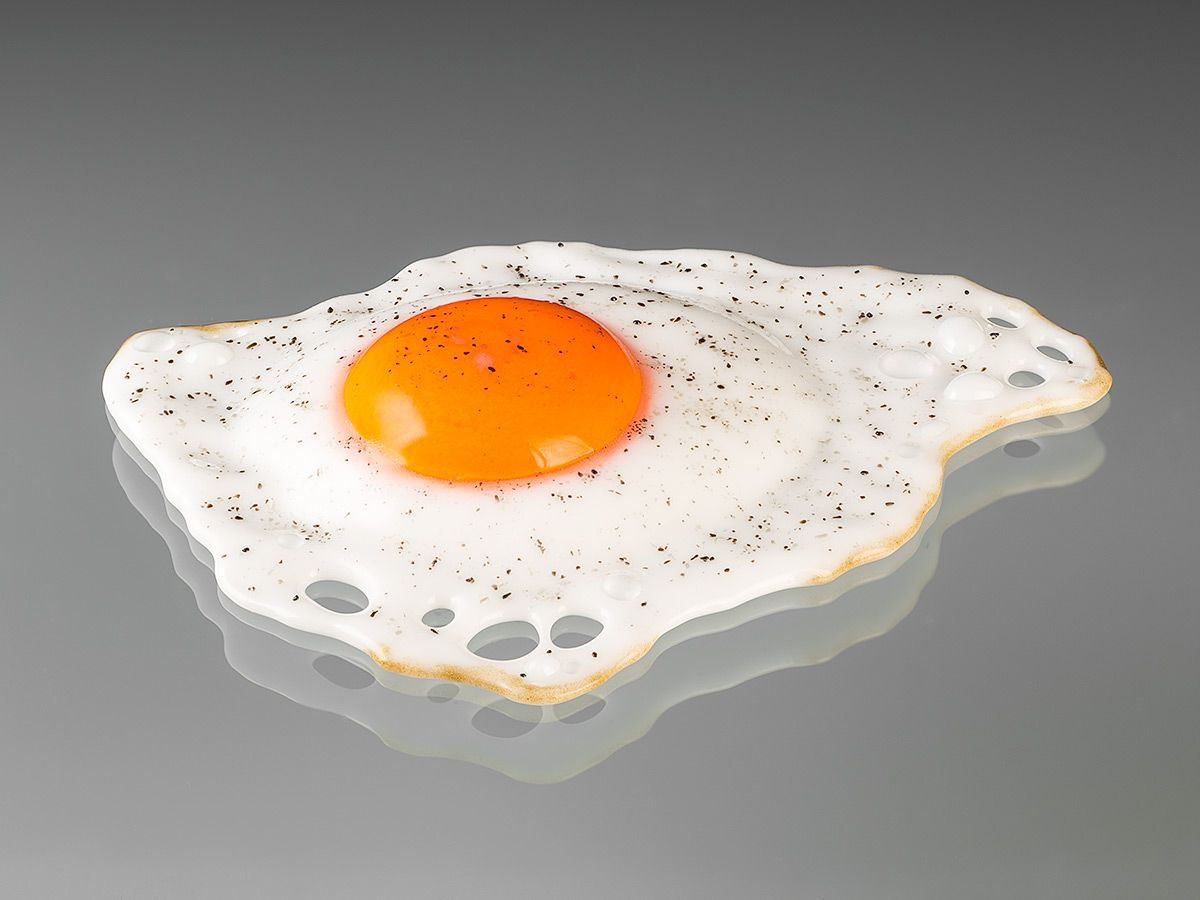The image displays a computer-generated fried egg, prominently positioned in the center against a gradient background that transitions from dark gray in the upper right to a lighter gray towards the lower left. The background features a silvery reflection of the egg, adding depth to the scene. The egg itself has irregularly shaped whites with puffy bubbles and some small holes, particularly near the browned, charred edges found toward the bottom and right, and slightly at the upper left as well. The yolk, a vibrant orange, is slightly off-center to the left, resting on a raised puff of egg white. Black or brown speckles of pepper are scattered across the surface, adding texture and flavor to the visual. The egg's reflection beneath it is notable, providing a double reflection effect that enhances the modern, minimalist aesthetic of the photograph.